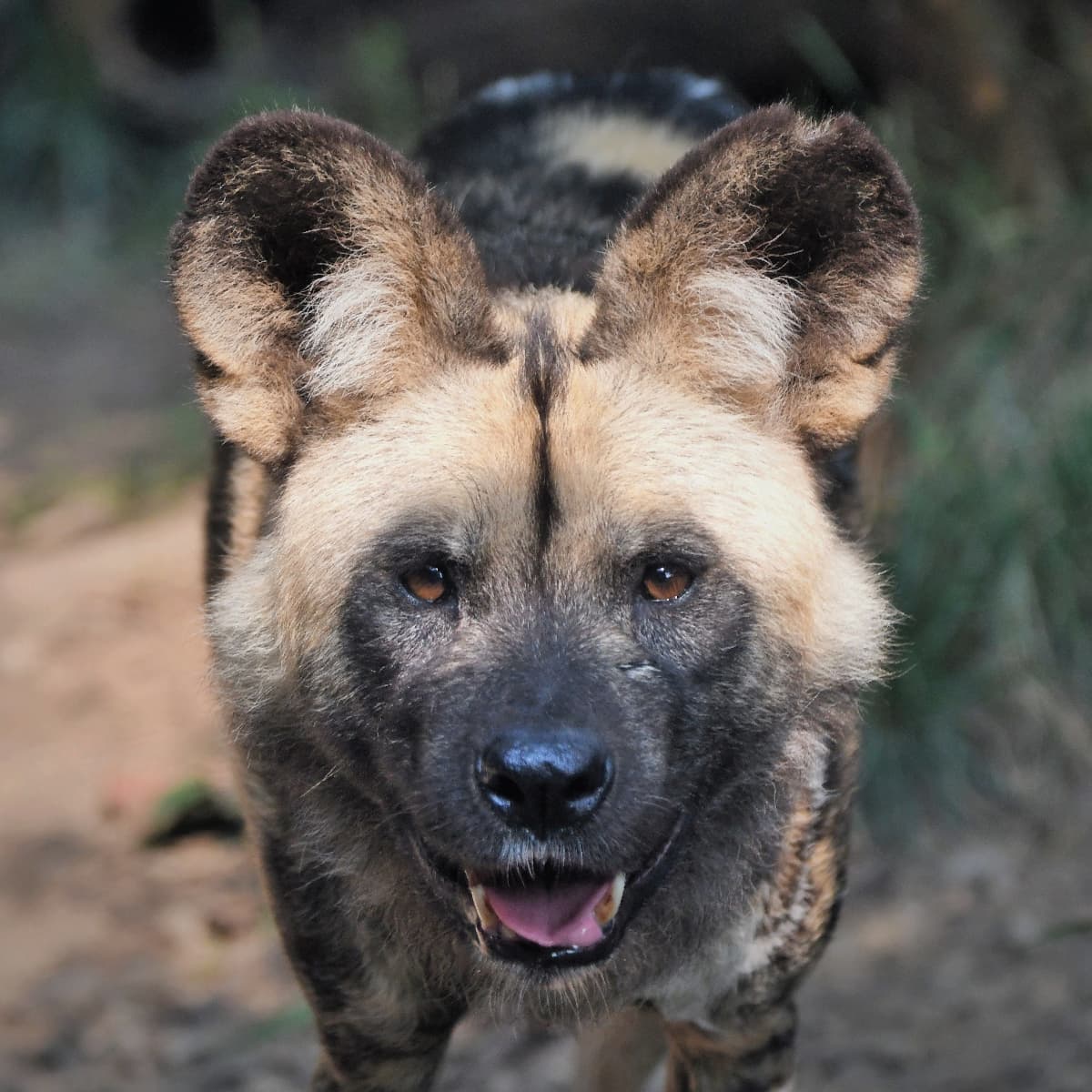This large square digital photograph provides a detailed close-up of the face of an animal, likely a hyena, though it has unique characteristics that might suggest a dog or a wolf. The creature's light beige fur, with blends of light, medium, and dark brown, forms an intricate pattern. Its ears stand upright but have a distinct rounded shape with white tufts in the middle, and there's a noticeable cut-out on the upper right ear. The animal's light brown eyes gaze directly at the camera, creating an intense, no-nonsense expression that almost evokes a sense of determination or anxiety.

Its black snout and nose stand out prominently, and its mouth is slightly open, revealing a pink tongue and yellowed canines on the bottom. A distinctive black vertical streak runs down the length of its forehead, partially dividing its predominantly light-colored face.

In the background, the blurred upper body of the animal blends into the image, showing patches of brown and black. The surroundings include blurred patches of dirt and grass, with browns dominating the left side and a mix of green and darker brown on the right. The overall color palette of the image is primarily brown and black, with slight hints of green.